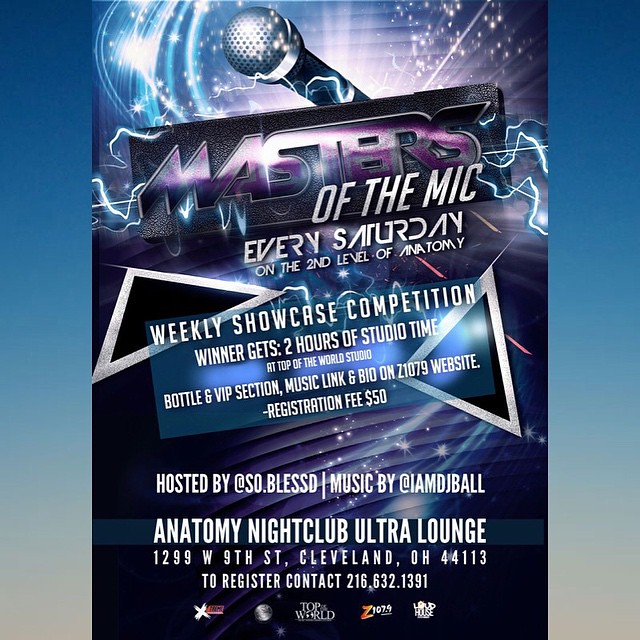This vibrant and eye-catching poster announces a musical competition event titled *Masters of the Mic*. Set against a dynamic background featuring shimmering blue sparkles, purple rays, and electric currents, the design evokes the atmosphere of a lively dance club. Central to the poster is a prominent silver microphone, highlighted with electric effects, symbolizing the event's musical focus.

The heading *Masters of the Mic* is written in a colorful, comic book-style font with "Masters" in a combination of purple and white, and "of the Mic" in a stylish silver font. The event is scheduled for every Saturday on the second level of the Anatomy Nightclub Ultra Lounge, located at 1299 West 9th Street, Cleveland, Ohio, 44113.

Below the heading, the center of the poster features a blue horizontal box that announces the weekly showcase competition. The winner of the competition will receive two hours of studio time at Top of the World Studio, along with a bottle and VIP section. More details, including music links and registration, can be found on the Z1079 website. The registration fee is $50.

The event is hosted by @so.blessd with music provided by @IAmDjBall. At the bottom of the poster, various sponsor logos, including Z107.9 and Loud House, are displayed in a row, solidifying the event's credible backing. For registration, contact 216-632-1391. This amalgamation of elements creates a lively and comprehensive invitation to an exciting weekly musical showdown.